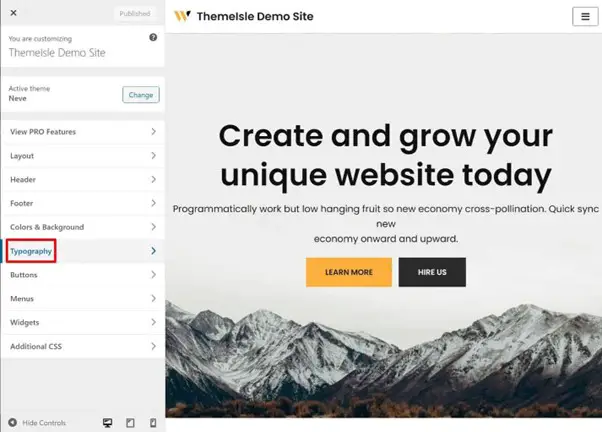The image showcases a promotional website banner with extensive details. On the right side, two diagonal yellow lines overlay a section that reads "THEMEISLE Demo Site." To the right of this area, an expansive mountain range covered in snow dominates the scenery. Below the mountains, a forest of low-lying trees in shades of brown, black, and dark green stretches across the bottom.

The central promotional text encourages users to "Create and grow your unique website today" and features motivational phrases like "Programmatically work," "Low-hanging fruit," "New economy," "Cross-pollination," "Quicksink," "New economy," and "Onward and upward." 

Beneath this text, a yellow rectangle with the call-to-action "Learn More" is prominently placed next to a black rectangle stating "Hire Us."

On the far left side, various categories are listed: "Typography"—highlighted in a red square—followed by "Buttons," "Menus," "Widgets," and "Additional CSS." Above the red square, more menu options include "Color and Background," "Footer," "Header," "Layout," "View," "PRO," and "Features."